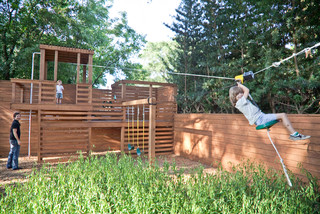In the image, a young boy is captured in mid-flight on a zipline set up in his own backyard. He is clad in a coordinated outfit of blue shorts, a blue top, and matching blue sneakers, and his long brown hair flows behind him as he holds onto the zipline. The zipline itself is yellow at the top, and a rope is visible hanging from the harness that secures him. He is suspended in the air, having started his thrilling ride from a large wooden play structure designed for children.

This play structure, built robustly from wood, serves as the launch point for the zipline. Inside this structure, up above, a younger sibling—possibly a little brother or sister—awaits their turn, cheering excitedly as they watch. Below, presumably the boy's father, dressed in jeans and a blue shirt, stands attentively, observing his son's adventurous ride with a watchful eye. The scene encapsulates a moment of joyful outdoor play and family togetherness.